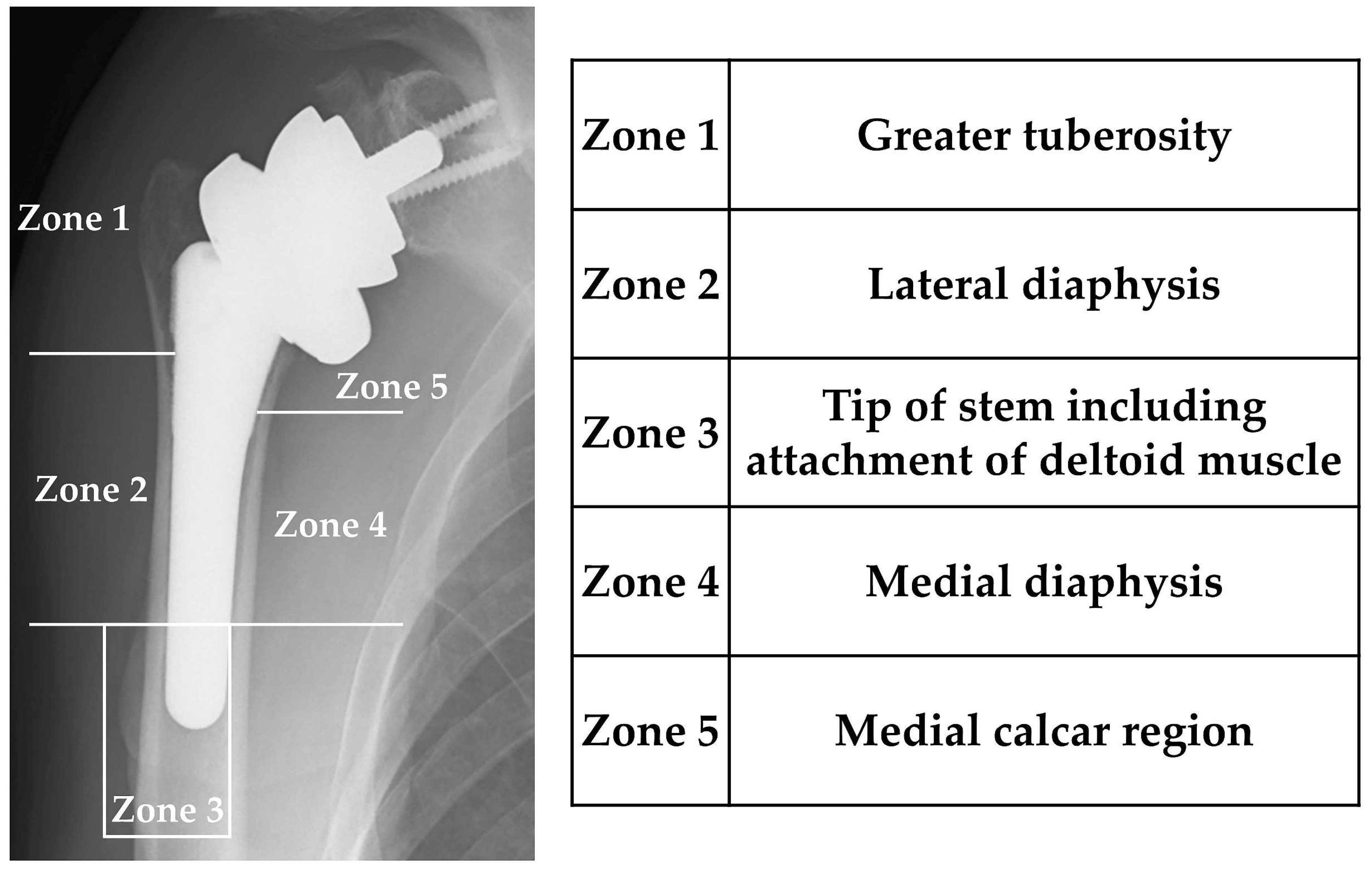The image features a detailed x-ray of a shoulder area, prominently displaying an artificial implant that replaces the natural shoulder bones. The x-ray, presented vertically on the left side of the image, is labeled with five distinct zones. Starting from the top, the zones are arranged as follows: Zone 1 at the top, Zone 2 beneath it, Zone 3 at the bottom, and Zones 4 and 5 on the right side of the image. Each zone is marked and named accordingly.

Adjacent to the x-ray on the right side is a table with a clear black border, containing two columns over five rows. The left column lists the zone names (Zone 1 to Zone 5), while the right column provides the corresponding anatomical or functional meanings:
- **Zone 1:** Greater tuberosity
- **Zone 2:** Lateral diaphysis
- **Zone 3:** Tip of stem including attachment of deltoid muscle
- **Zone 4:** Medial diaphysis
- **Zone 5:** Medial calcar region

The text within the table is written in black against a white background, offering clear explanations of the zones depicted in the x-ray.